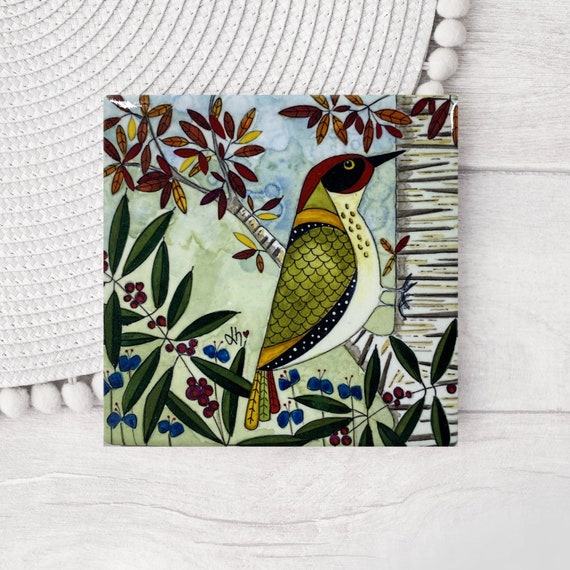This is a detailed image of an abstract painting depicting a bird that closely resembles a woodpecker. The bird is perched on a white tree trunk, with distinctive black and yellow stripes, that looks like it might be a birch. The bird itself has a striking appearance: a red head, a black band across its eyes resembling a bandit mask, a white chest and neck, and green and yellow wings with red wingtips. Surrounding the bird are intricate details including limbs with richly pigmented leaves in red, orange, and yellow, along with red berries and blue flowers. The background features a blue sky and possibly watercolor swirls of blue-green hues. This artwork sits atop a white wooden table, covered with a white woven table runner or circular tablecloth adorned with small puffballs along the edges. An initial, possibly "LH" or "DH," is visible slightly off-center on the left side. The entire scene is set against a background that includes more blue leaves at the bottom, enhancing the vivid and lively atmosphere of the painting. The image is portrayed against a contrasting backdrop, such as the edge of a carpet or rug, further framing this colorful and detailed piece of art.